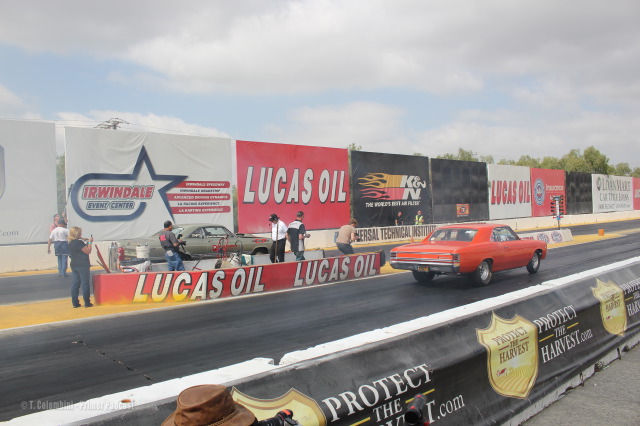The image depicts a bustling outdoor racetrack set against a backdrop of pale blue sky, dotted with wisps of clouds and the tops of some trees. Dominating the scene are two racing cars: an orange car actively driving on the track from the bottom left to the middle right, and a gray car undergoing a pit stop attended by a crew of about six people. In front of the dynamic orange car, a barricade features a prominent gold shield with the black lettering "Protect the Harvest" and a black banner proclaiming "ProtectTheHarvest.com." Surrounding the action, a lively crowd of spectators can be seen in the background, adding to the atmosphere of a professional racing event. Prominent branding and sponsor logos are visible throughout; large signs include a big red "Lucas Oil" advertisement and a neighboring white sign with a blue star reading "Irwindale Event Center." Additional, less distinct ads line the billboards bordering the track. Toward the middle left of the image, a woman captures the scene with a photograph, encapsulating the vibrant energy of the racetrack. The colors of the cars stand out vividly against the surrounding elements, creating a dynamic and engaging composition.